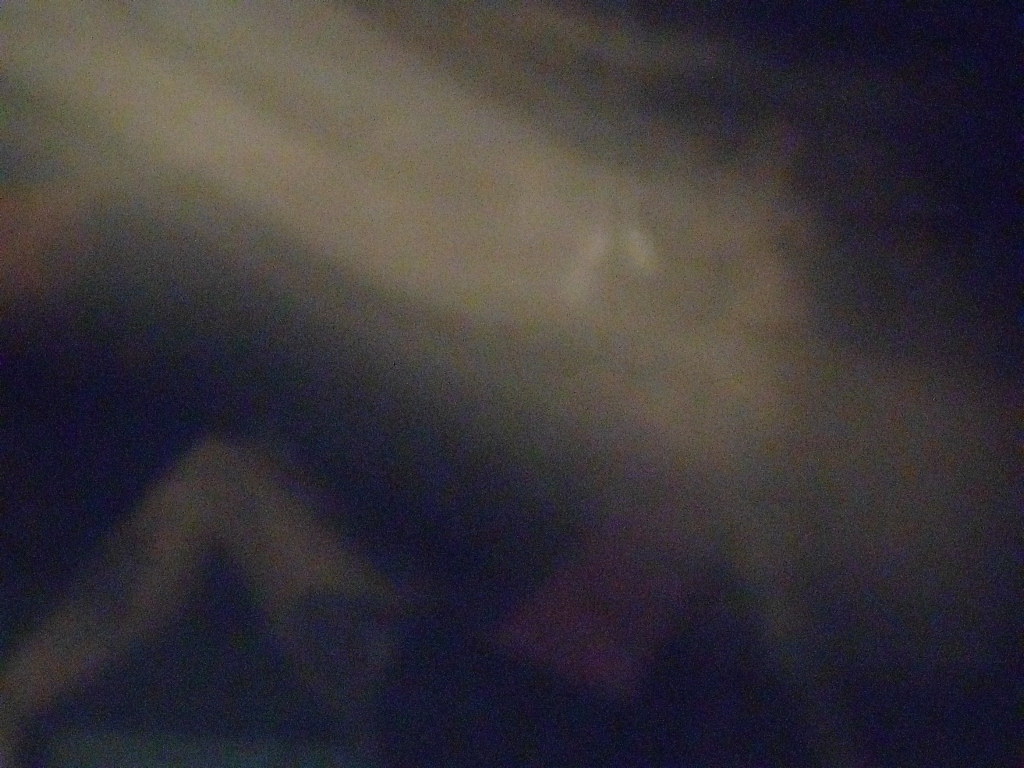This grainy and abstract image features several color blobs that create an enigmatic scene. Dominating the composition is a large, light tan brushstroke that extends from the top left to the middle right of the frame, giving an impression of movement. The top right corner and the lower part of the image are shrouded in black, adding to the mystery. A reddish-colored rectangle stretches from the lower middle to the middle right, evoking a sense of structure amidst the chaos. In the bottom left corner, a tan triangular shape, resembling a bent leg, adds a human-like element to the otherwise amorphous picture.